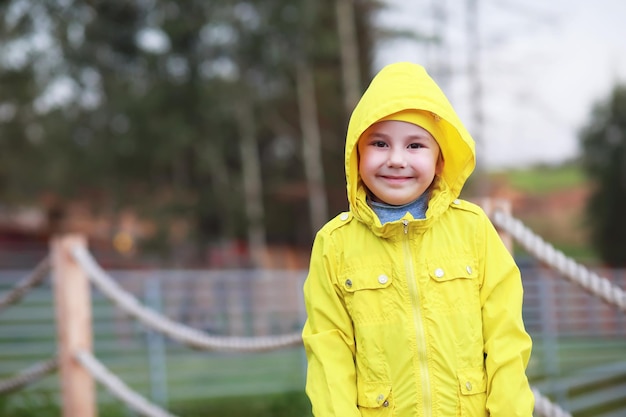This photo captures a young child, likely a pre-teen, smiling warmly and facing the camera. The child is slightly off-center to the right, presented from the waist up. They are dressed in a bright yellow raincoat that appears new, with a hood covering their head, concealing their hair. Visible underneath is a gray turtleneck or undershirt. The raincoat, zipped up all the way, features at least four pockets, two on each side of the chest.

The blurry background reveals an overcast sky with a light gray hue in the top right corner, and tall trees on the left. Directly behind the child is a wooden post with thick ropes threaded through, creating a guardrail or barrier. Further back, there is a tall, sturdy metal fence with horizontal rails. The overall setting indicates a daytime outdoor scene, where the focus remains sharply on the child's cheerful expression amidst the slightly obscured natural and structural elements behind them.